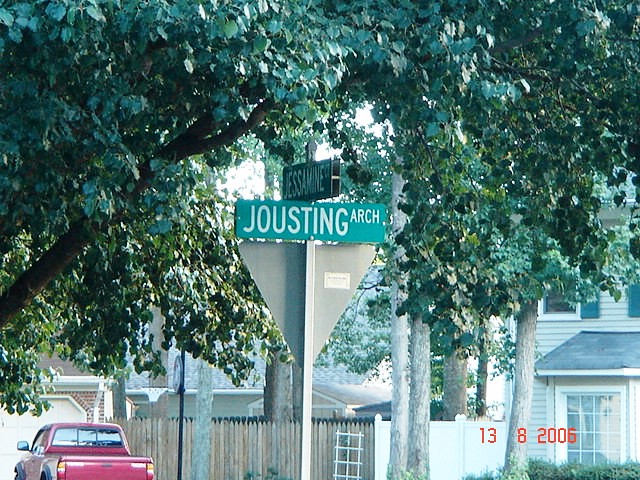The photograph, dated August 13, 2006, features an overexposed scene marked by a red timestamp in the bottom right corner. Dominating the foreground is a signpost, viewed from behind, revealing an upside-down triangular yield sign. Mounted above this yield sign is a street marker reading "Jousting Arch." Perpendicular to this, another sign indicates "Jessamine." The background is filled with an assortment of trees, adding to the suburban setting. Additionally, a red pickup truck is parked nearby, and a fence lines the area, with several houses visible in the distance.